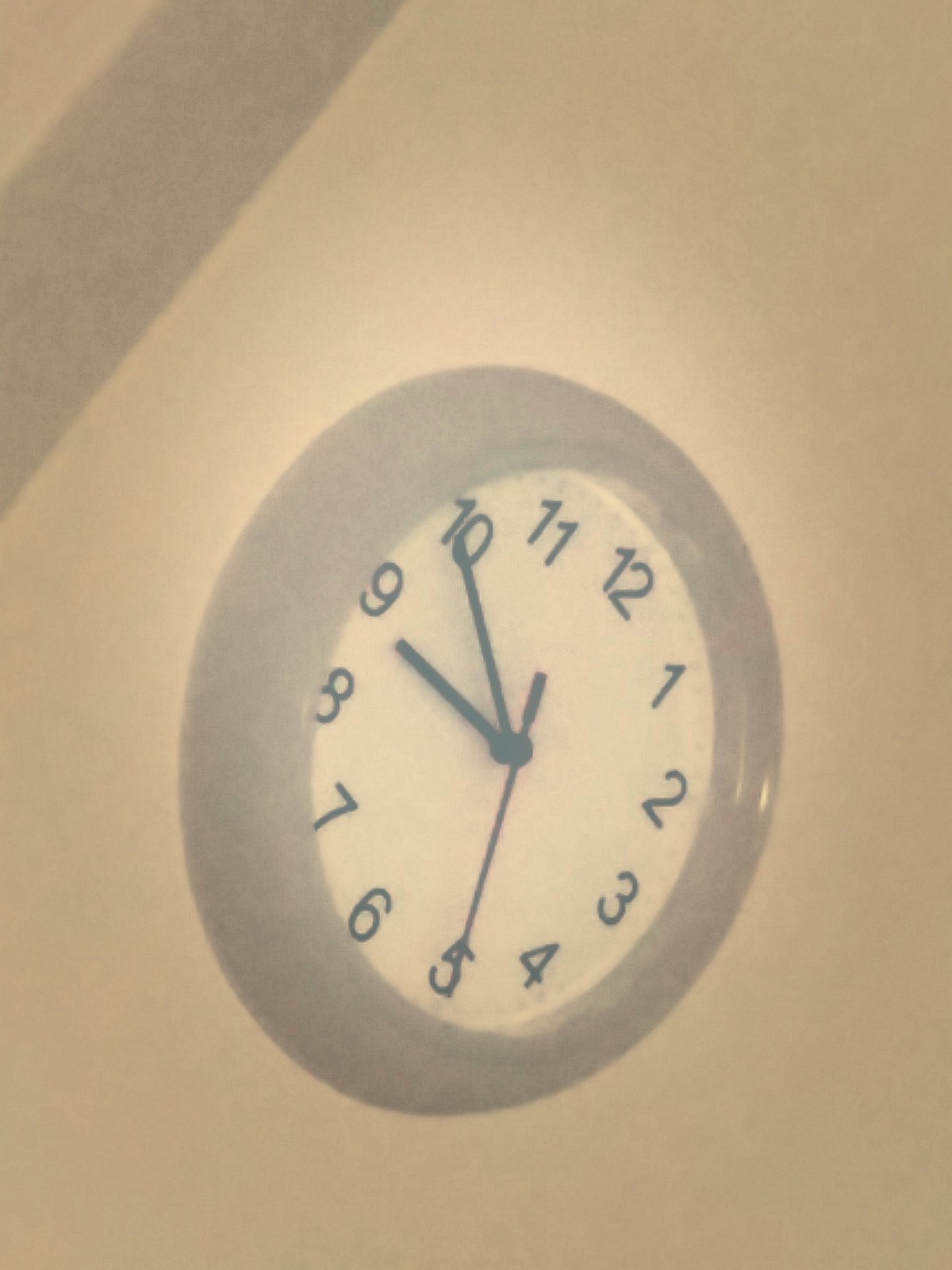In this photograph, taken under low light conditions with a noticeable foggy ambiance, a round clock affixed to a white wall is prominently featured. The clock is slightly tilted to the right, causing the number 12 to shift from its upright position. It has a gray plastic case that carries a slight reflective gleam on the side. The clock's face is white, adorned with bold black numbers, and it is equipped with three black hands—an hour hand, a minute hand, and a second hand—neatly held together at the center by a black screw. The time displayed on the clock is 8:49.